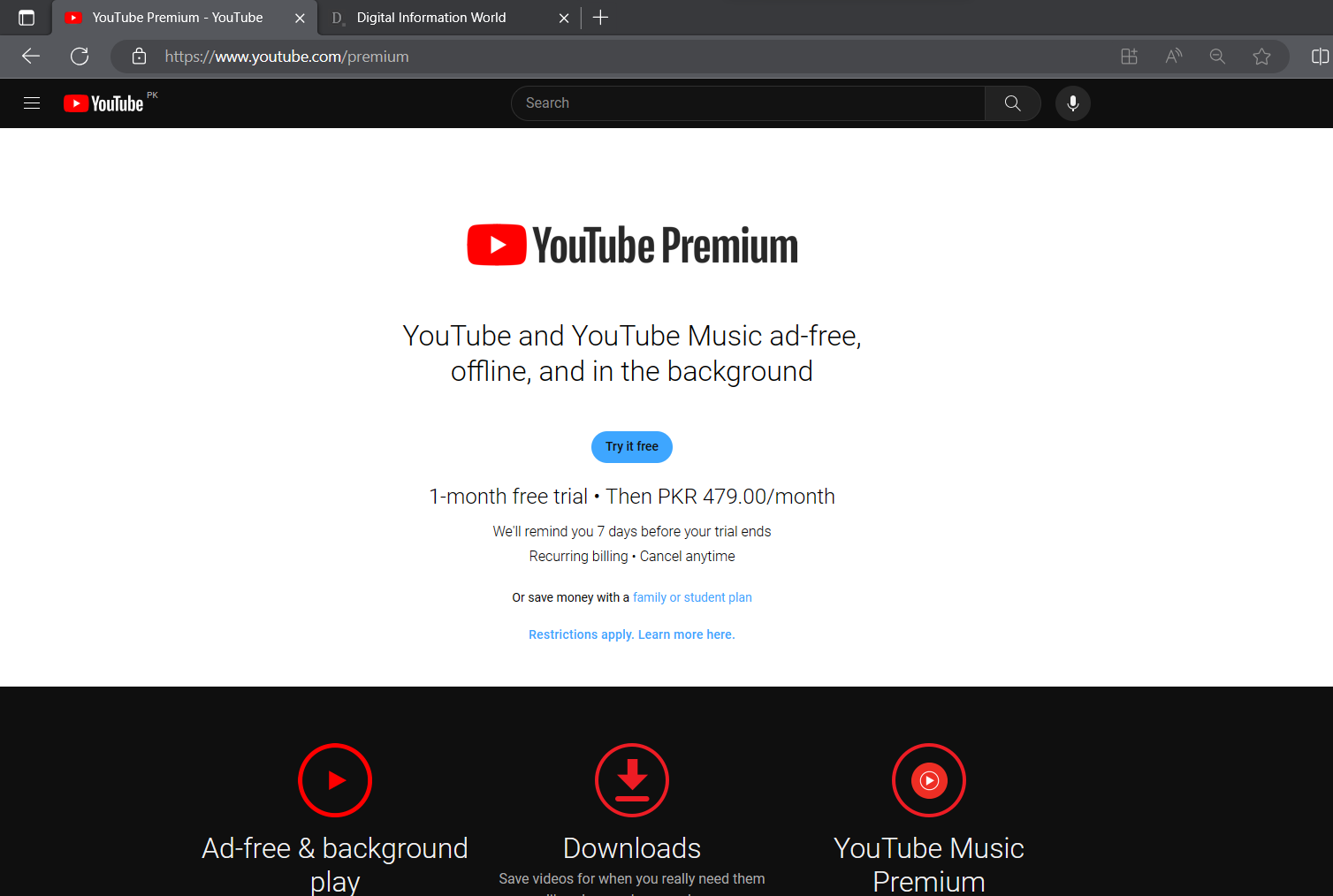The rectangular image, oriented horizontally, depicts an open webpage in a web browser featuring YouTube Premium. At the top of the page, the URL clearly displays "youtube.com/premium." A black navigation bar contains the YouTube logo on the left, a hamburger menu icon adjacent to it, a search button in the center, a user icon to the middle-right, and a microphone icon on the far right.

Beneath this, a predominantly white section features prominently a red rectangular box with a white play triangle icon and the text "YouTube Premium." The text below reads, "YouTube and YouTube Music ad-free, offline, and in the background." Further down, a blue oblong button invites users to "Try it free," followed by text that offers "One month free trial," with a subsequent cost of "PKR 4.79 a month." Additionally, it notes, "We'll remind you seven days before your trial ends. Recurring billing, cancel anytime."

At the bottom of the webpage is a black section highlighted by three red circles, each accompanied by descriptive text. The left circle denotes "Ad-free and background play," the center one indicates "Downloads," and the one on the right specifies "YouTube Premium Music."